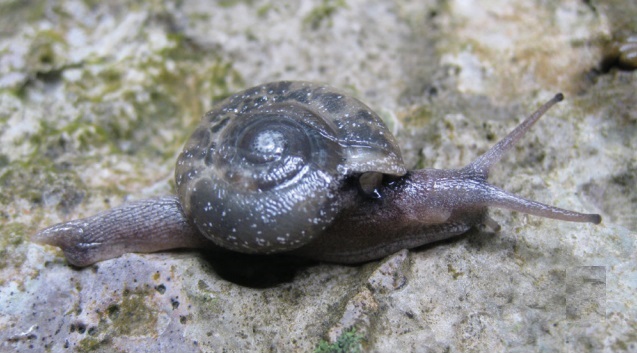This detailed photograph captures a close-up view of a snail on a white, rocky, textured surface. The rock features specks of green, which could indicate moss or mere discoloration, alongside gray and black markings. Central to the image, the snail’s shell—spiraling in a form reminiscent of a cinnamon roll—is a striking tan taupe with dark brown and black patterns. The snail’s body, extending from beneath the shell, is a captivating pinkish-gray with a subtle translucence and a sparkling sheen. Two prominent antennae jut outward from the snail’s head in a V-shape, with their tips notably dark. A faint shadow cast by the shell enhances the textural depth of the rocky surface, accentuating the snail’s serene traversal.